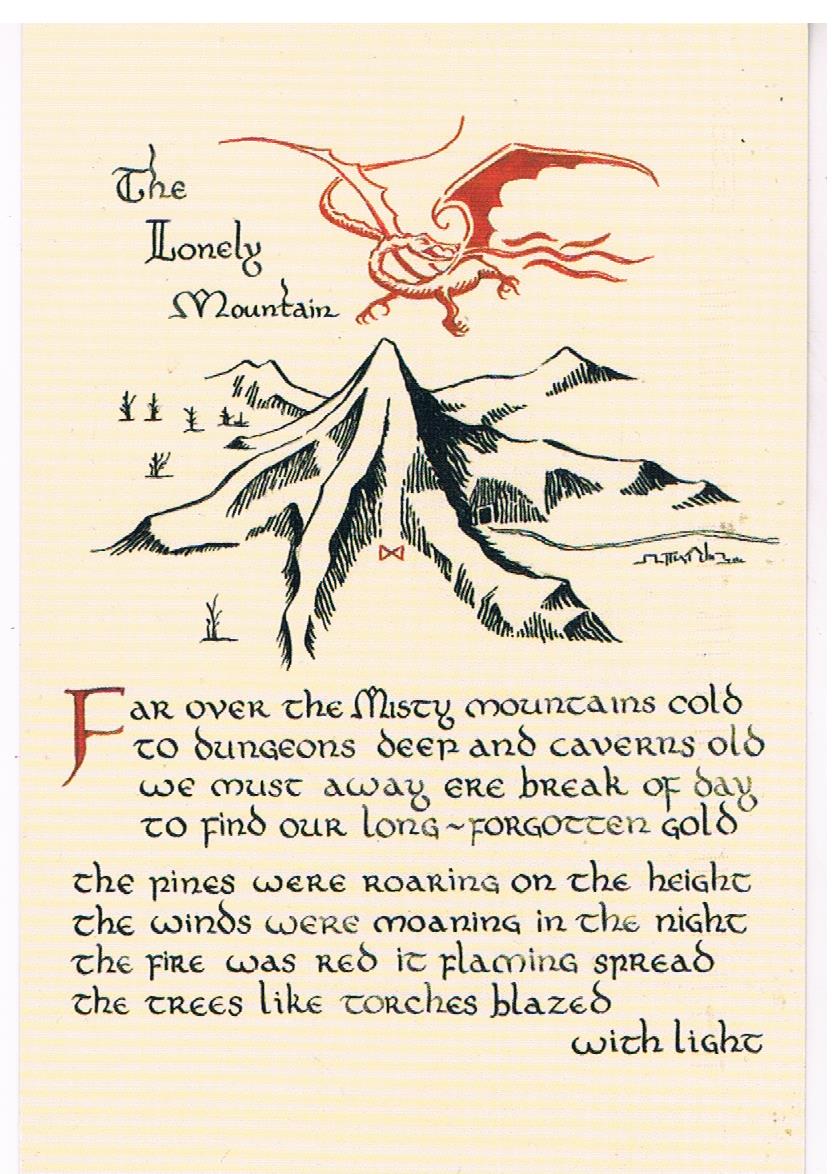This image appears to be a photograph of a beige page showcasing an artistic piece. It prominently features an elaborate red dragon flying over a sharp mountain peak, which is depicted with a mix of black and white areas to signify snow coverage. The mountain is surrounded by barren trees or bushes.

In the upper left corner, the words "The Lonely Mountain" are inscribed in a fancy, old-timey calligraphy script. Below the dragon and mountain illustration, a poem is written in an old-world font, starting with a large capital "F" in red, while the remaining text is in black. The poem reads:

"Far over the misty mountains cold
To dungeons deep and caverns old,
We